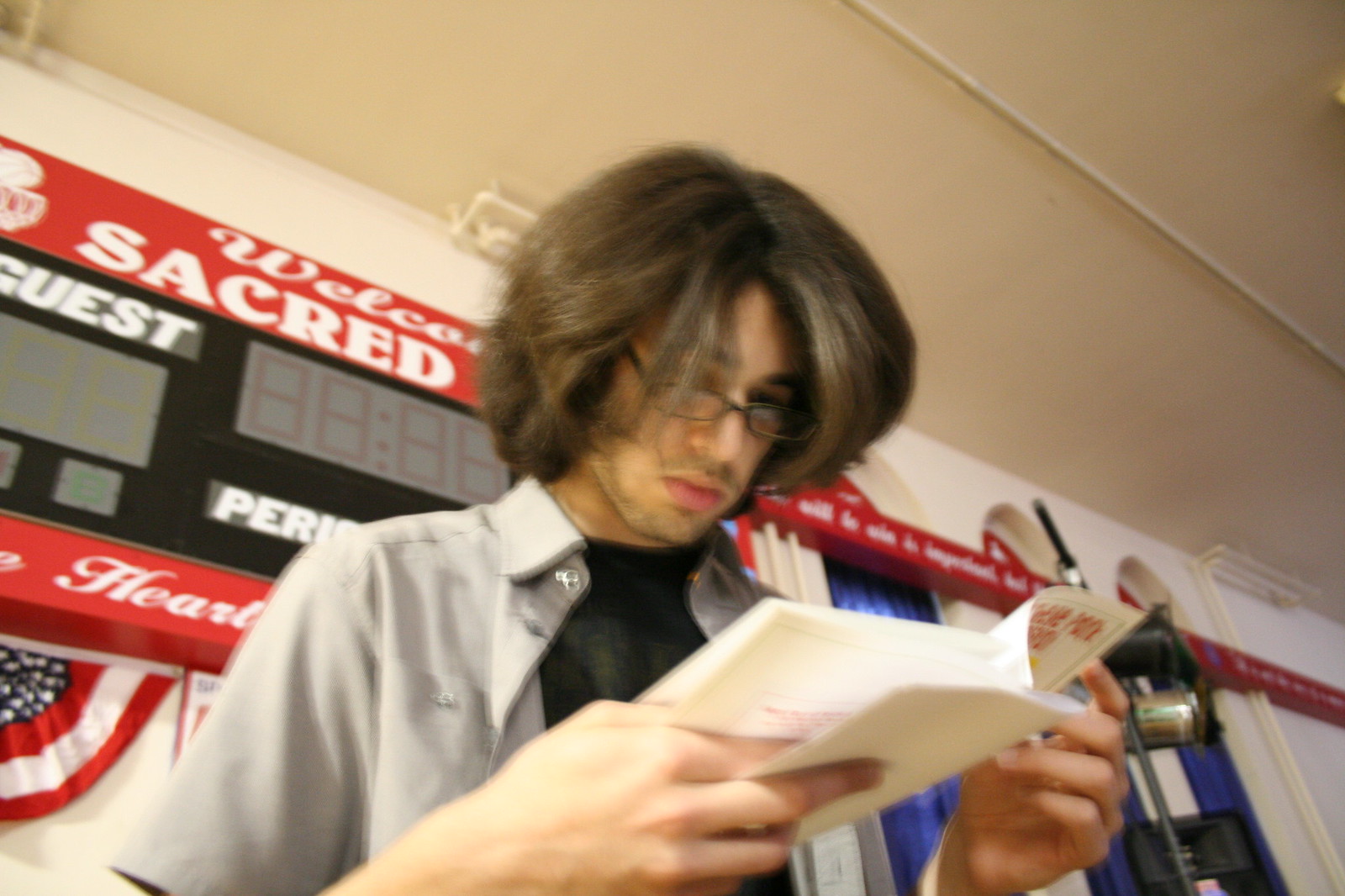This photograph captures a young man with light skin and long, poofy brown hair that falls to his chin, partially covering his ears. He has a stubbly beard and wears glasses. The man is dressed in a black t-shirt underneath an open, short-sleeve light bluish-gray button-down shirt. He is looking down intently at a white pamphlet or program with red text, which he holds in front of him. The background reveals that the scene takes place in a gymnasium, as indicated by a large scoreboard mounted on the pale yellow wall behind him. Above and below the scoreboard, red banners with white text can be seen, one of which partially reads, "Welcome Sacred." The image is somewhat blurry and unfocused, emphasizing the brightly lit wall more than the man himself.